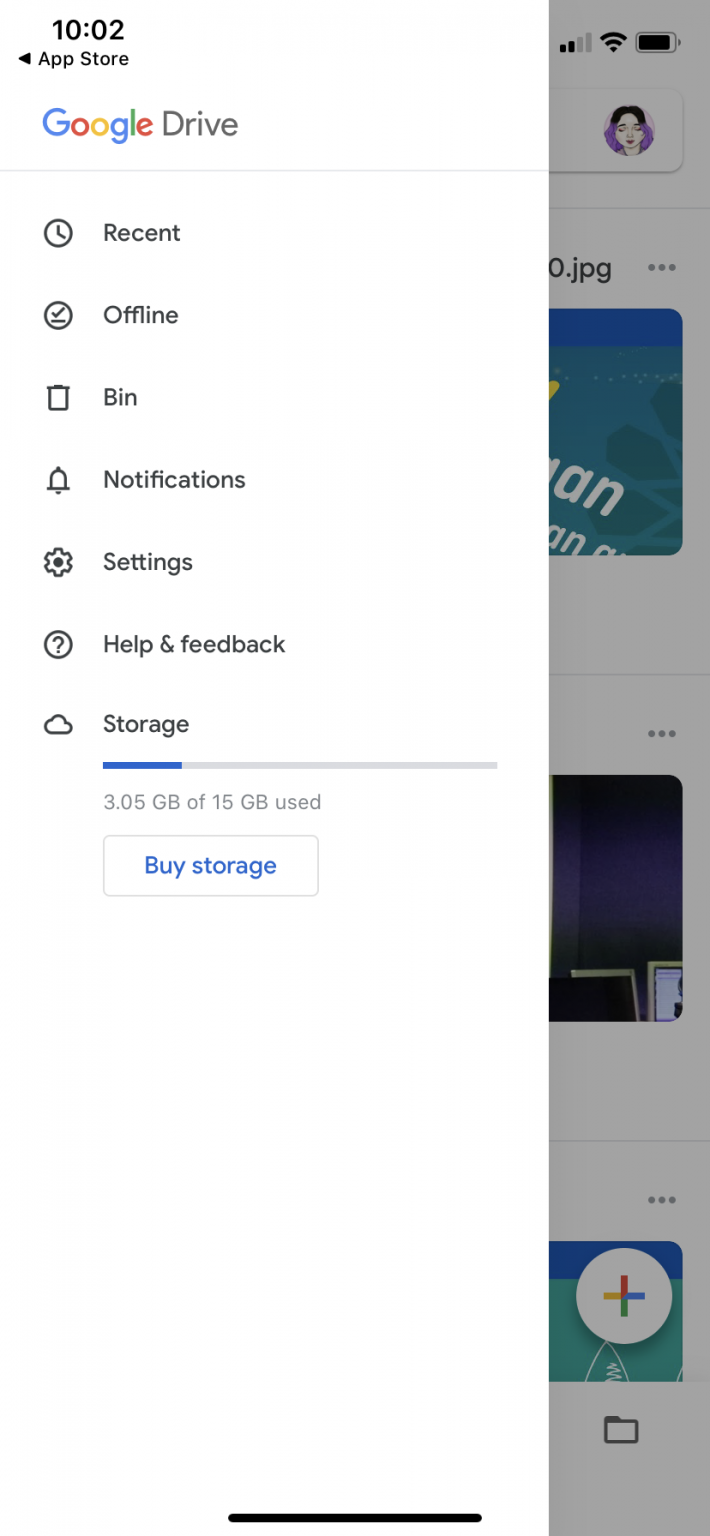The image is a screenshot taken from the App Store displaying the Google Drive application interface. The timestamp at the top shows 10:02. Below the timestamp is a faint gray line separating the time from the app content. 

In the main interface, there is a clock icon next to the word "Recent." Below, there is a series of menu options, each with its own icon. The first is a checkmark inside a circle labeled "Offline." Next, an icon resembling a pot with a lid is labeled "Bin," followed by a bell icon labeled "Notifications." Further down, a gear icon signifies "Settings," and a question mark inside a circle indicates "Help and Feedback." Lastly, a cloud icon marks the section for "Storage."

Under the "Storage" section, a progress bar shows usage: a blue line partially filled, transitioning into gray, indicating 3.05 GB of 15 GB used. Below the progress bar is a "Buy Storage" button highlighted in blue text.

At the bottom right corner of the screenshot, a partial view of the phone's status bar is visible, showing the battery life at approximately 95%. The edge of other icons can also be seen, although they are partially cut off.